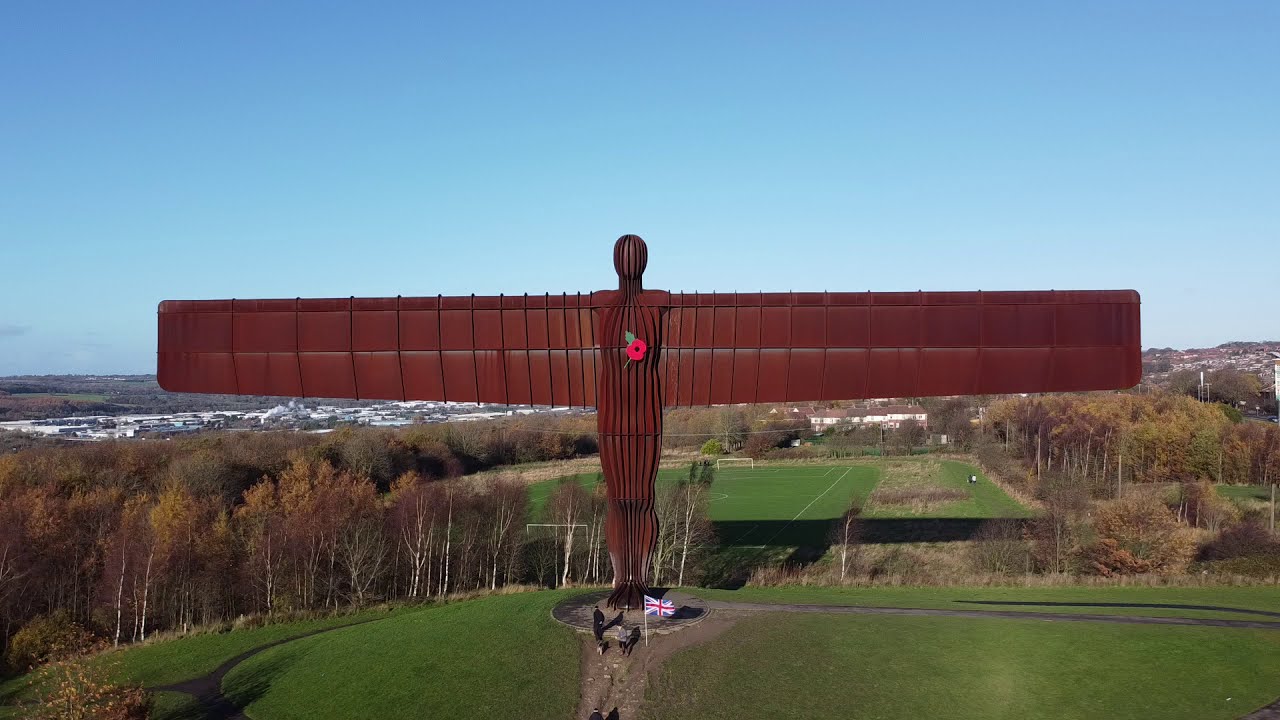The photograph, taken on a bright, cloudless day, captures a sprawling outdoor scene dominated by a massive, copper-colored or rusty-red statue crafted from sheet metal or wire. The statue, a striking humanoid figure resembling a woman with discernible curves, features arms that resemble airplane wings. Over its chest, where the heart would be, is a prominent red or pink flower. The base of the statue grounds a Union Jack (British flag) fluttering in the breeze, with a couple of people nearby, their details blurred by the statue's colossal presence. The statue stands on a gently sloping hillside, bordered by vibrant, green grass and a walking path that curves in from the right. Beyond the statue, a large soccer field stretches out, flanked by a row of houses in the distance. The top half of the image is filled with a clear, azure sky, adding to the serene backdrop. The photograph's composition, captured from an elevated, possibly drone perspective, showcases both the grandeur of the sculpture and the idyllic surroundings, epitomizing realistic, representational drone photography.